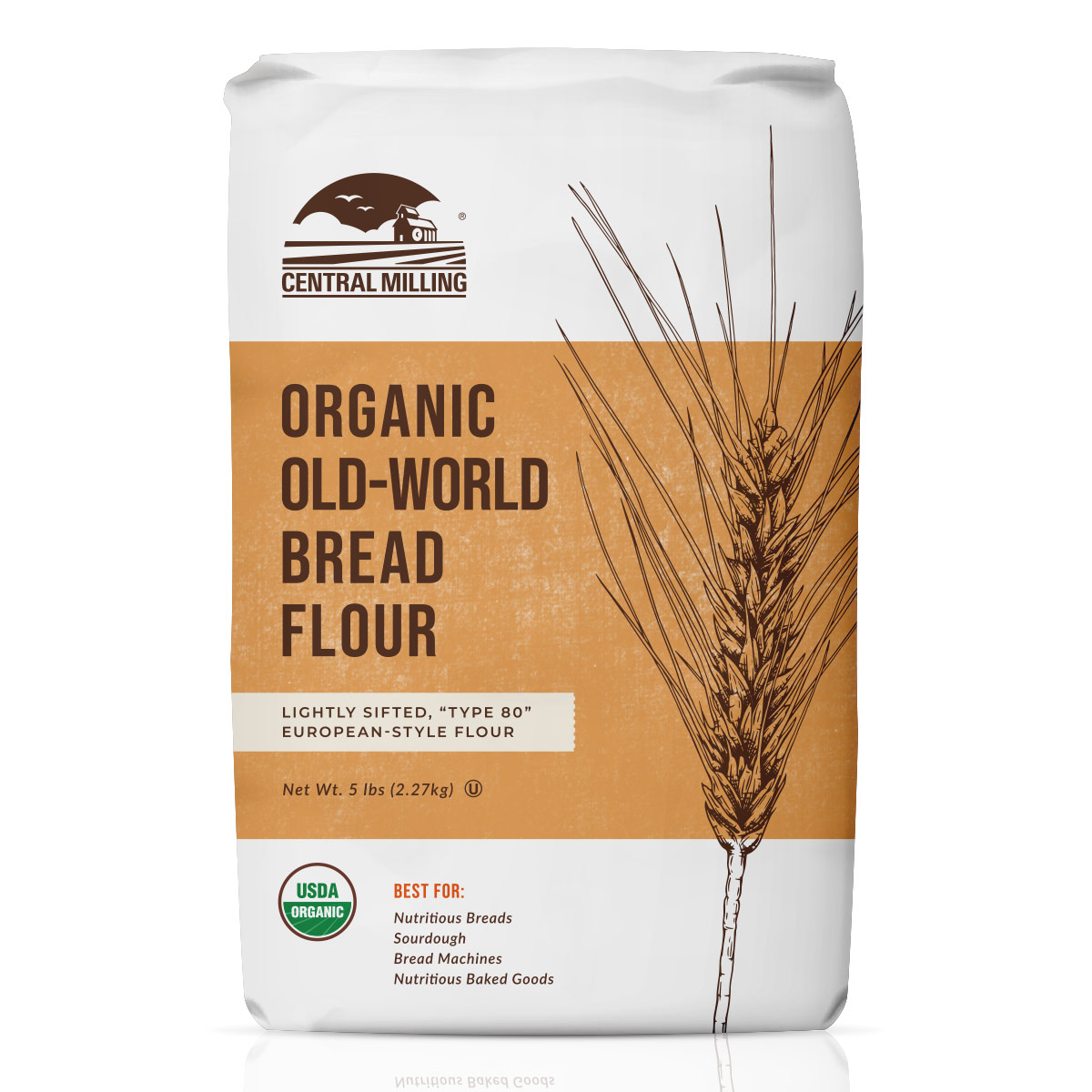The image showcases a meticulously designed bag of flour set against a stark white, semi-reflective surface, creating the illusion of it floating in a white void—perfect for an online product listing. The bag is distinctively divided into three sections: white on the top and bottom, and tan in the center. An elegant black outline of a wheat plant spans the entire height along the right side. On the left, a variety of logos and texts adorn the package. 

At the top left, the logo for "Central Milling" is printed in brown, accompanied by a charming hand-drawn image of a farm, complete with a barn, sunshine, and two white birds set against a brown sky. Below this imagery, on the tan section, bold black text reads "Organic Old World Bread Flour." Further down, a small white rectangle contains brown text that states "Lightly Sifted Type 80 European Style Flour." 

Additionally, the bag states the net weight in brown text as "5 pounds 2.27 kilograms." A USDA organic certification logo, featuring a black outline and colored half in green and half in white, is situated in the bottom left corner. Adjacent to this, orange and brown text declares the flour "Best For: Nutritious Bread, Sourdough, Bread Machines, Nutritious Baked Goods." The detailed product design underscores its organic and premium quality, making it a visually appealing and informative choice for consumers.